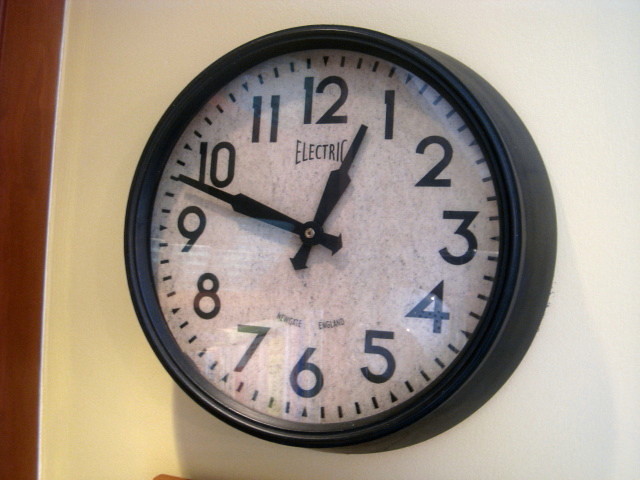The image features a large, round analog clock with a black housing, prominently displayed on an off-white wall. The clock's face is a marbled mix of white and gray, detailed with black numbers and hands, as well as a small silver fastener at their center. Above the numbers 5, 6, and 7, the words "NEWGATE ENGLAND" are clearly visible, while "ELECTRIC" appears in bold black letters just below the number 12. The clock's clear glass cover reflects some light, adding a subtle shine to its surface. To the left, the image includes a glimpse of a brown-toned partition or wall, providing a contrasting background that emphasizes the clock's striking presence. The short hand of the clock is positioned near the 1, while the long hand is two notches below the 10, indicating the current time. Black increment marks around the clock's face further enhance its detailed and precise design.